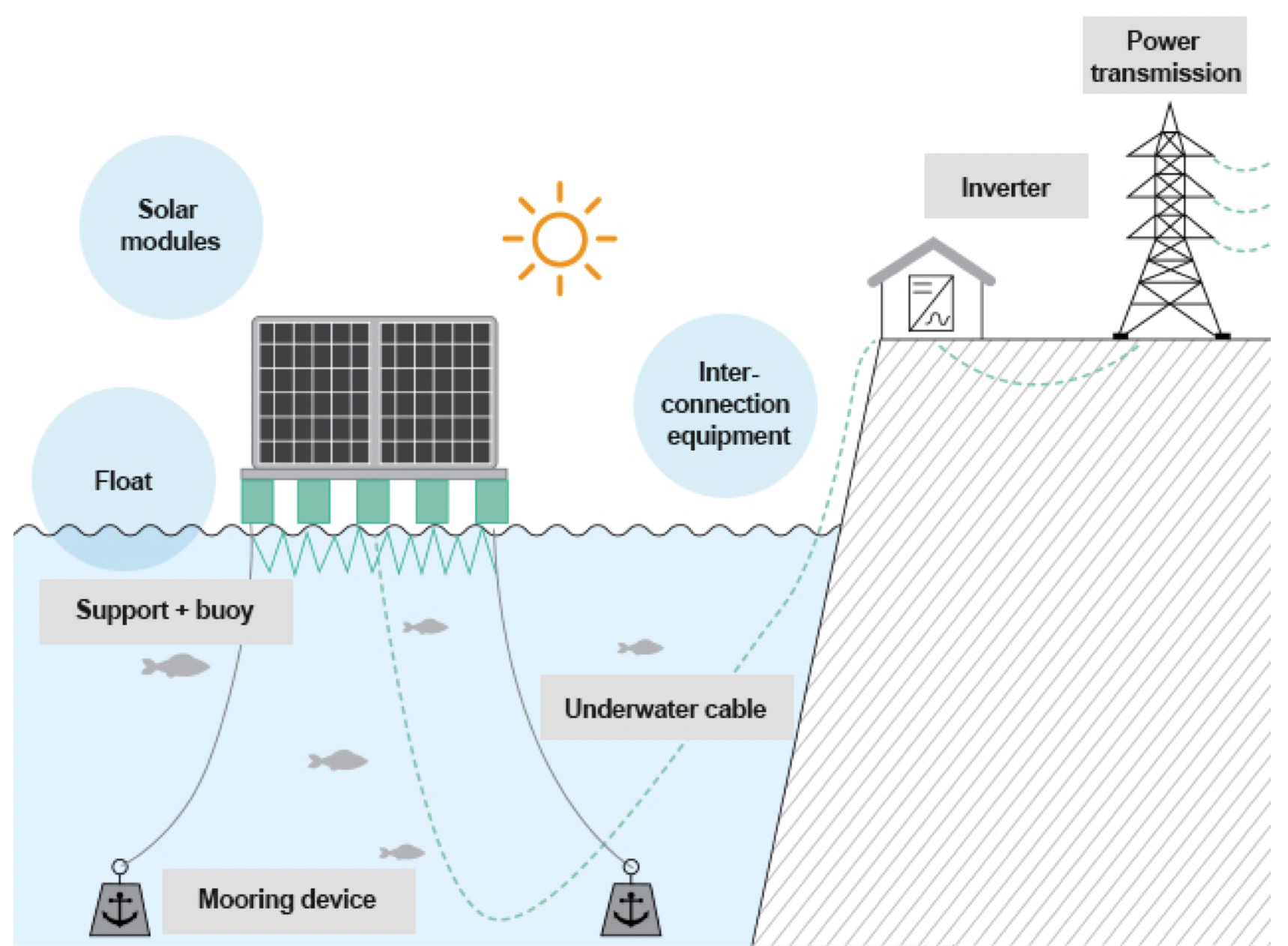The diagram illustrates a solar energy collection system integrated with a water body, designed in a simple, corporate-style manner often found in instructional manuals. On the left, floating solar modules, depicted as black and gray grids, rest on teal-colored flotation devices in a large body of water, possibly the ocean. The sun, shining from above, provides the necessary solar energy. 

Underneath the solar modules, there are mooring devices and support buoys ensuring stability. An underwater cable extends from these floating structures toward the shore. The cable connects to interconnection equipment positioned at the water's edge, indicating a transition from the floating solar array to land.

On the right-hand side of the diagram, atop a cliff-like formation rising from the water, a small house-shaped building marks the location of the inverter. This inverter converts the collected solar energy into usable power, which is then transmitted via a high-voltage power line, depicted as a large power transmission tower. This entire setup showcases the journey of solar energy from collection in water to transmission on land.